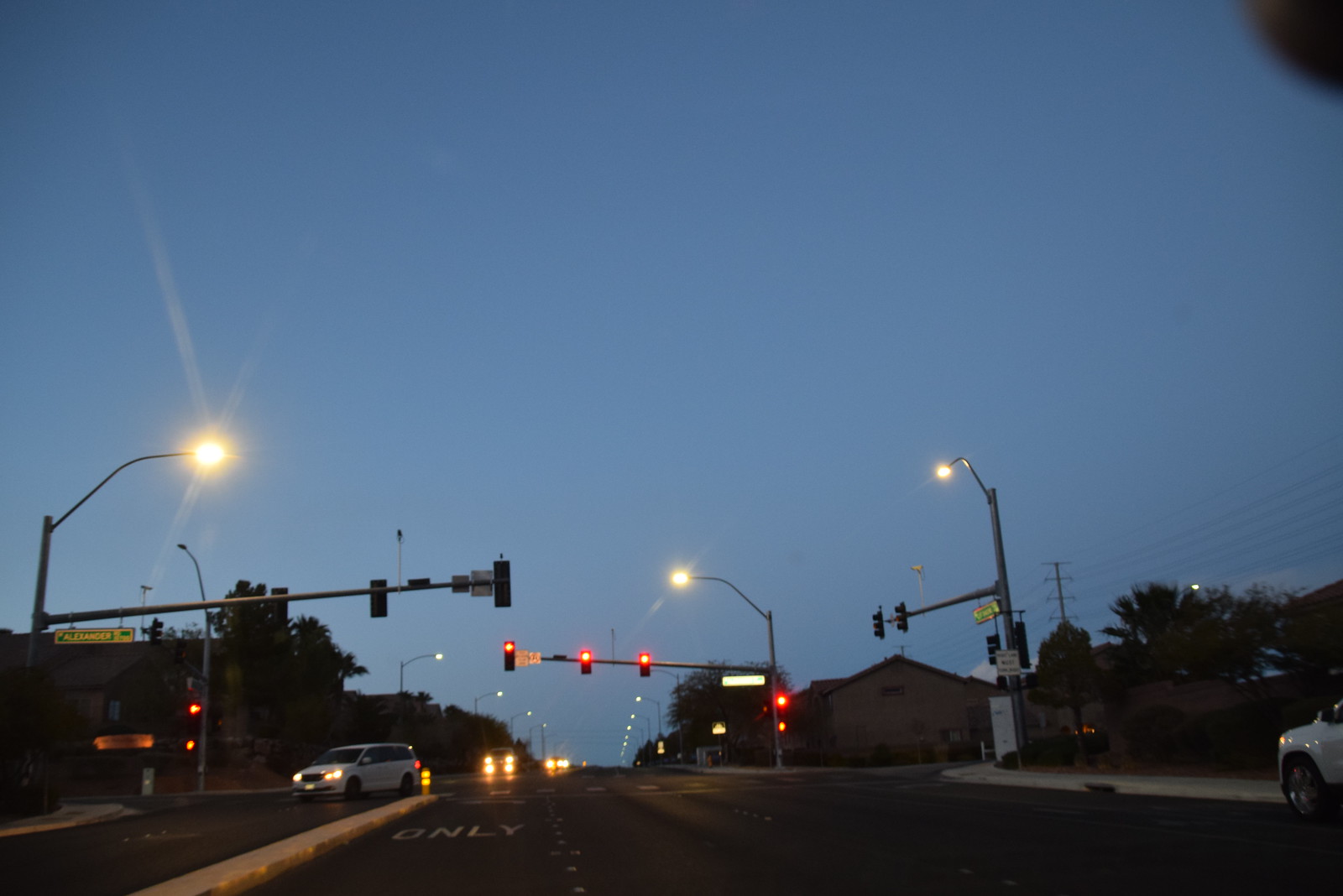A nighttime photograph captures a scene from a moving vehicle driving down a dimly lit road. The sky is dark, but it is not pitch-black, suggesting early night. In the distance, a red traffic light hangs, casting a soft glow on the intersection below. Multiple streetlights illuminate the road, creating a dotted line of light that recedes into the horizon.

Silhouettes suggest the presence of trees, their leaves rendered indistinct by the darkness. The moon appears faintly in the sky, adding a celestial touch to the otherwise urban scene.

On the left side of the road, a white minivan is visible, making a left turn at the intersection. On the opposite side, the oncoming headlights of other vehicles glimmer in the distance, contributing to the lively yet serene atmosphere.

Light streaks, indicative of the photo being taken in motion, add dynamic lines to the image, reminiscent of how lights appear to someone with astigmatism. The road is marked with the word "ONLY" and a right-turn arrow, guiding traffic. A crosswalk is faintly visible, though the area appears devoid of pedestrians. The overall image is surprisingly clear despite the movement, capturing both the stillness and motion of a night drive.